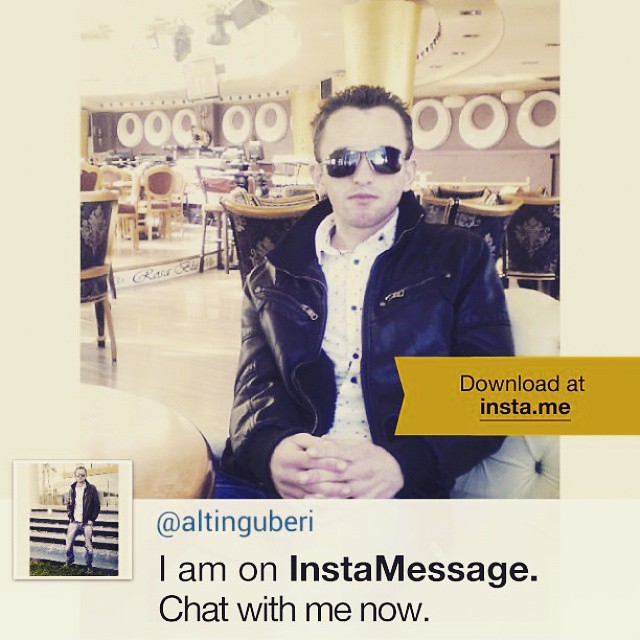The image is a promotional advertisement featuring a man, likely in his early thirties, with short brown hair and a widow's peak. He exudes a suave and cool demeanor, wearing sunglasses, a black leather jacket, and a white button-up shirt. The man is seated with his hands clasped in his lap, in what appears to be a light purple-hued room, possibly a restaurant or nightclub, adorned with random white ring decorations and a noticeable gold column behind him. The primary photo of the man is bordered by a tan frame, and a secondary, smaller image of him, wearing the same attire, is situated at the bottom left. His Instagram handle "at Alton Guberi" is displayed in blue beneath the main image. Superimposed on the central photo is a ribbon-like background with text urging viewers to "download at insta.me." Additional black text states, "I am on InstaMessage, chat with me now," suggesting an invitation to engage with him on the InstaMessage app.